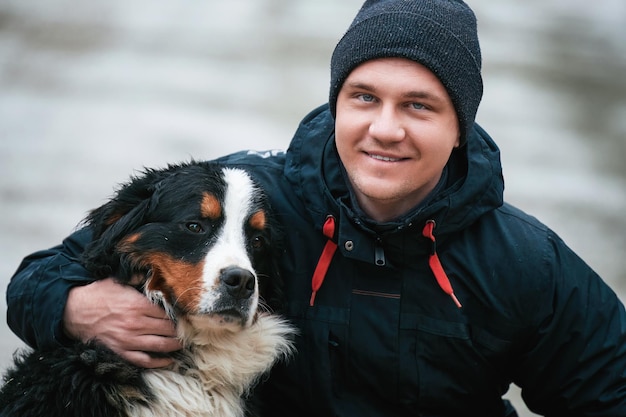This is a detailed color photograph of a smiling Caucasian man, likely in his thirties, and his dog. The man wears a dark knit cap and a black parka with a hood, which features prominent red shoelace-type drawstrings. His hood is not up; instead, it rests around his neck. The man's arm is affectionately wrapped around his dog, which appears to be a Bernese Mountain Dog. The dog is comfortably cuddled up to the man's shoulder, with both of them looking directly at the camera, though only the man is smiling.

The dog’s face has a unique coloration: a white stripe runs down its forehead to its nose, the muzzle is white with some brown near the mouth and eyebrows, and the dog's cheeks also show brown patches. Additionally, the dog's chest is predominantly white, flanked by black on either side. Both man and dog are shown from the chest up, making it unclear whether they are sitting or standing. The blurred background hints at cold weather, suggested by the man's warm attire, but it is indistinct, leaving the setting ambiguous.